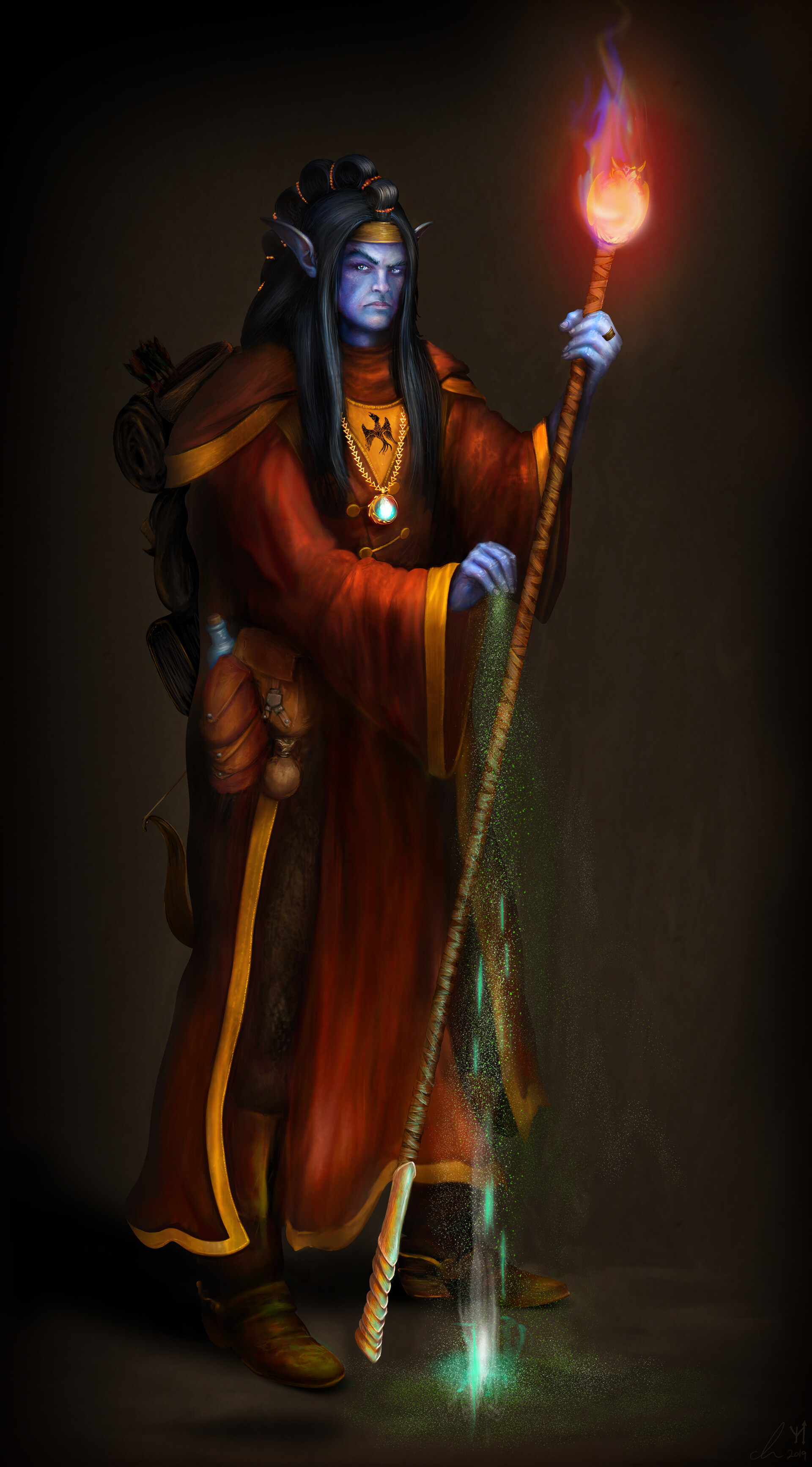This cartoon, possibly computer-generated, portrays a tall figure with neon blue or purplish skin, reminiscent of a video game character. The character stands at the center of the image against a dark, somewhat brownish and non-detailed background. He has pointed ears akin to an elf and long black hair styled half up and half down, with a gold headband and small buns running along the top. Wearing a long robe that transitions from brown to reddish hues with yellow and gold trim, his attire is intricate and detailed.

The figure wields a long staff that extends from his feet to slightly above his head, emitting an almost fiery glow with red flames and purple tinges. Additionally, his other hand appears to be conjuring a green, sparkly beam, possibly suggesting the opening of a portal. Adorning his chest is a detailed black emblem, potentially representing a bird or dragon, while a glowing blue amulet hangs from a gold chain around his neck. His outfit is complemented by yellow-brown boots and various accessories, including a backpack, satchels on his right side, and a canister or container on his hip. The complete absence of text highlights the vivid use of colors such as black, red, blue, silver, and brown, bringing the animated figure to life in this compelling scene.